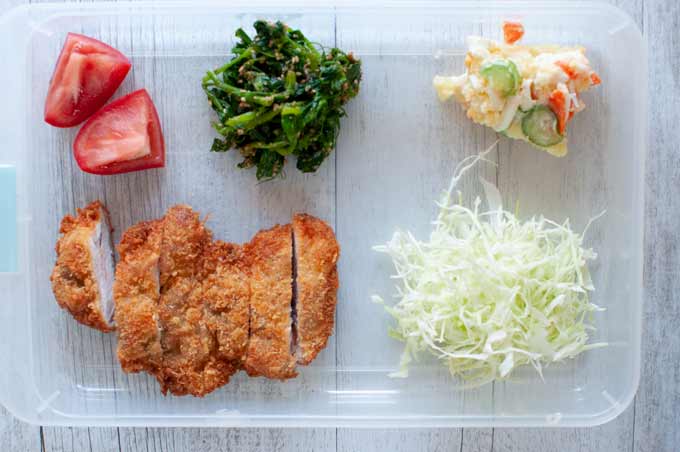The photograph showcases a clear plastic tray of food set atop a whitewashed wooden table. The tray contains a breaded and sliced chicken cutlet, positioned at the bottom left, revealing its crispy exterior and tender meat. Adjacent to the cutlet is a finely shredded raw cabbage slaw. Moving clockwise, the top left section houses two tomato wedges. To their right, in the top middle, sits a serving of cooked greens, likely collard greens or spinach. The top right compartment features what resembles a cracker topped with a spread of red and yellow, possibly cheese or dip, garnished with green peppers or cucumbers. This assorted meal, arranged with precision to keep foods separate, creates a simple yet detailed presentation.